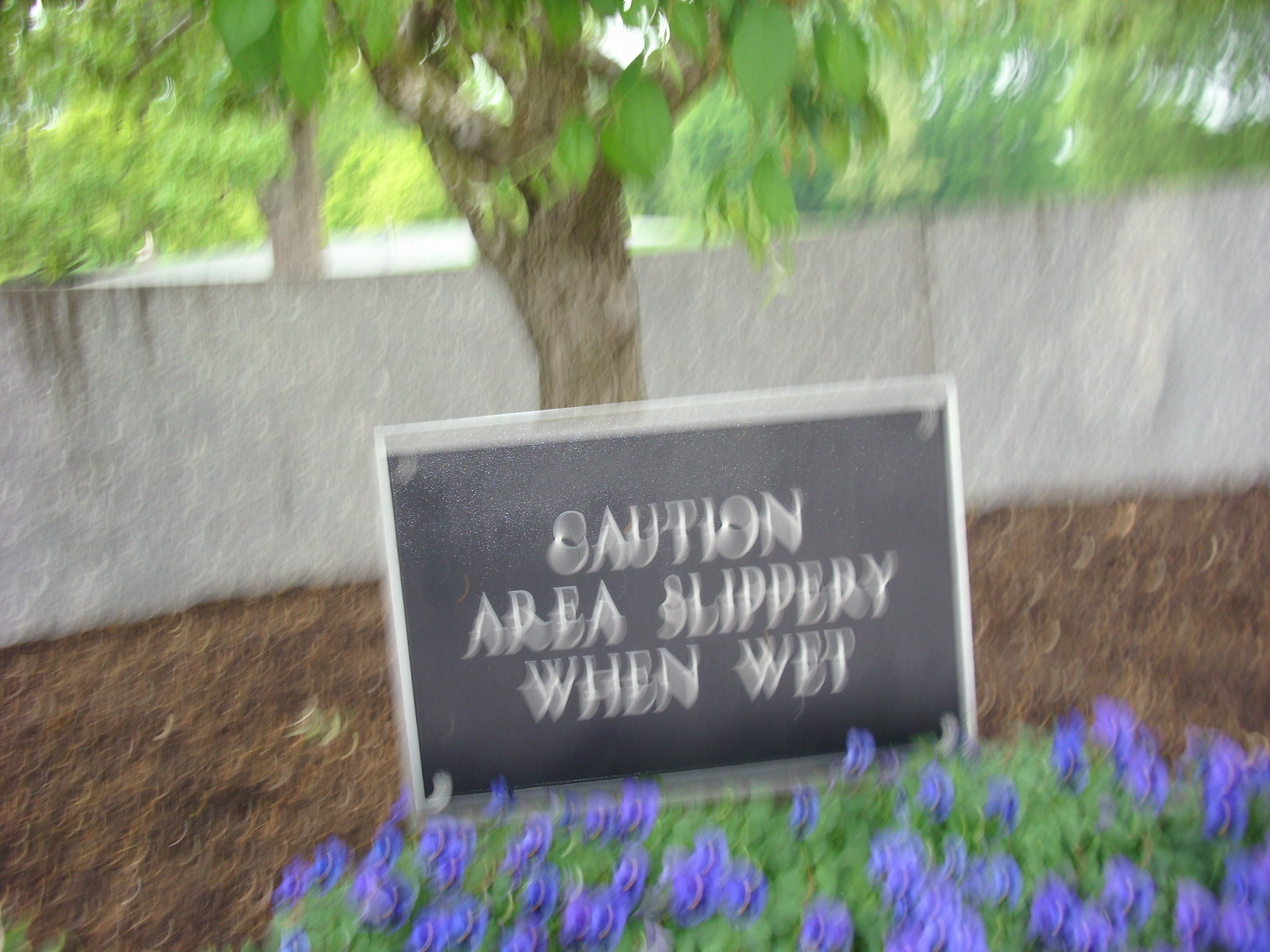In this image, a slightly out-of-focus photograph captures a black and white caution sign warning of a slippery area when wet. Despite the blurriness, the details behind the sign are discernible. Dominating the background is a rather large tree with a robust brown trunk and numerous sturdy branches, all adorned with an abundance of green leaves. Encircling the tree is a heavy, solid grayish-white gate that provides an element of security. In the foreground, the ground is covered in a rich layer of brown mulch, interspersed with vibrant violet and green flowers that add a touch of color and liveliness to the scene.